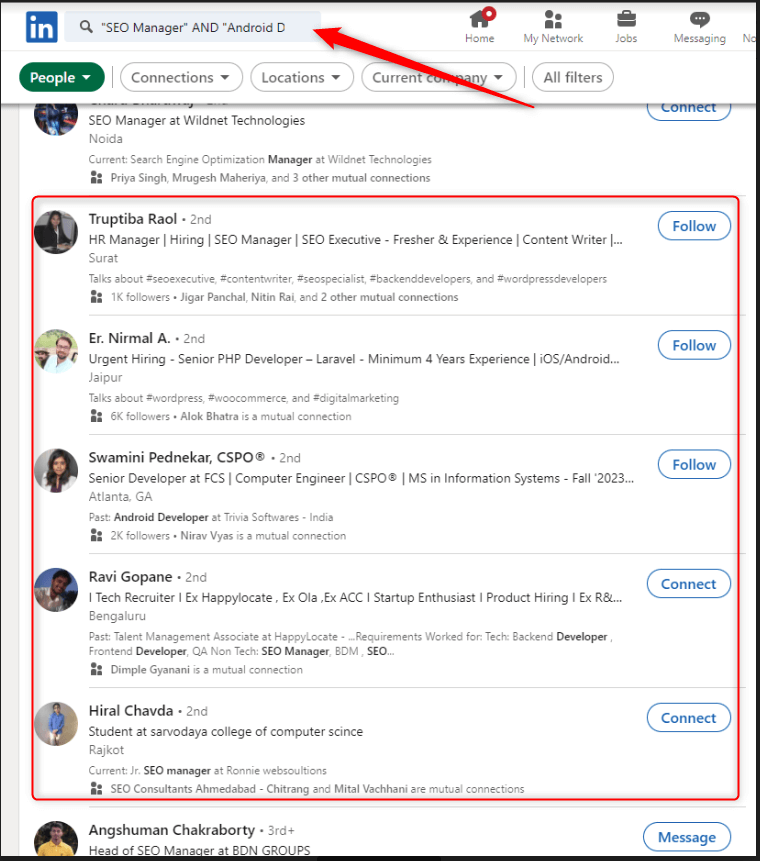In the upper left corner of the image, a blue square contains the letters "IN." Beside this, a search bar displays the text "SEO Manager" and "Android" in quotations. A red arrow extends from the right side of the word "Android," pointing back and slightly downward. To the left of this, the word "People" is enclosed in a green circle, with a small arrow pointing downward. 

A large red square outlines a section featuring five different profile pictures aligned to the left. The first profile picture is dim, making it difficult to see, but it is apparent that the person is wearing a blue shirt. The name associated with this profile is "Tripita Raul, HR Manager." Below this, there is an image of a man with black hair and glasses named "Ernirmala." Next, a woman with dark brown hair appears to be wearing a white doctor's jacket, identified as "Swamini Pednekar." Finally, at the bottom, there is an image of a person in a blue shirt and white pants, named "Hiral Chavda."